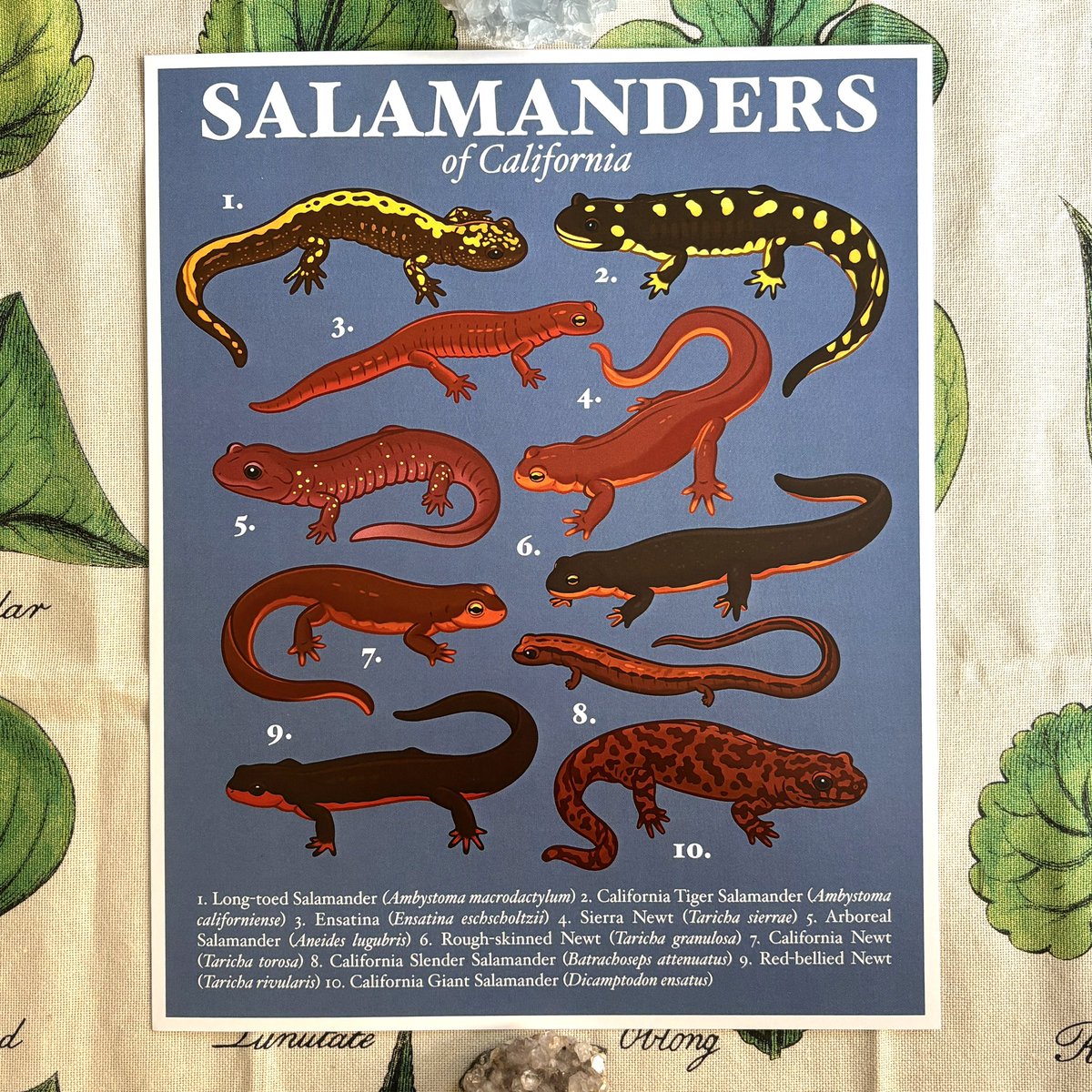This close-up photograph showcases a rectangular paper poster set against a light tan fabric background adorned with green leaf illustrations. The poster, bordered in white and featuring a dark blue background, prominently displays the title "Salamanders of California" at the top, with "of California" in smaller white print below "Salamanders." The central focus is on ten finely detailed images of salamander species, each labeled with a white number from 1 to 10. At the bottom of the poster, a footnote lists the common and scientific names of each species. Specifically, the salamanders include:

1. Long-toed Salamander (Ambystoma macrodactylum), brown with a yellow back.
2. California Tiger Salamander (Ambystoma californiense), dark brown with gold specks.
3. Ensatina (E. eschscholtzii), small and reddish-orange.
4. Sierra Newt (Taricha sierrae), slightly larger with a reddish-orange back and light orange underbelly.
5. Arboreal Salamander (Aneides lugubris), dark red in color.
6. Rough-skinned Newt (Taricha granulosa), dark brown with an orange underbelly.
7. California Newt (Taricha torosa), brownish-red back with a light red underbelly.
8. California Slender Salamander (Batrachoseps attenuatus), long, thin, and tiny red.
9. Red-bellied Newt (Taricha rivularis), stout with a black back and a red belly.
10. California Giant Salamander (Dicamptodon ensatus), tubby light red with dark brownish-red blotches.

A small grayish-white stone is placed at the bottom of the image. The diverse coloration of the salamanders ranging from reds and browns to blacks and yellows is vividly captured, emphasizing the rich biodiversity of California's salamander species.